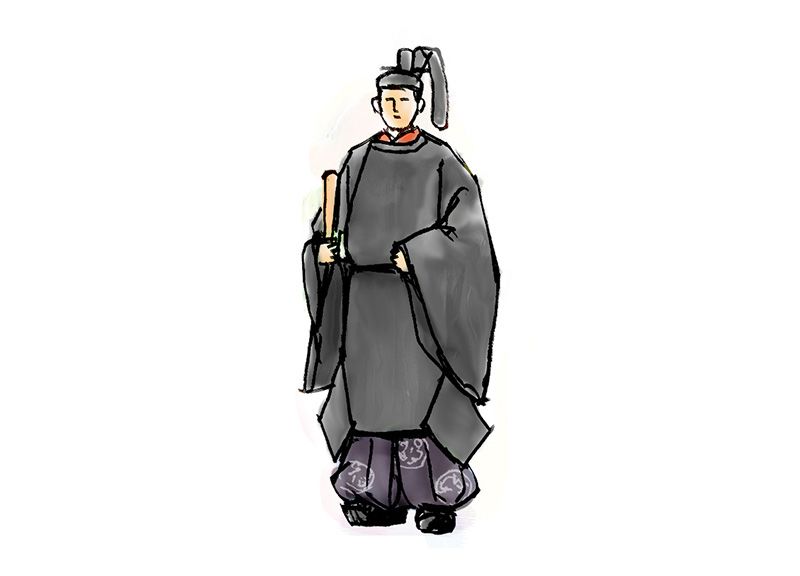This detailed watercolor drawing portrays an Asian male character with very fair skin, reminiscent of a monk or a graduate in traditional attire. Set against a white translucent background, he wears a dark gray robe over a red shirt and a belt around his waist. His gray, puffy pants contrast with his similarly gray, puffy shoes. The character's intricate headpiece, an extension of his gray hat, curves and bends down to his right shoulder, adding an elaborate touch to his attire. In his right hand, he holds what appears to be a cream-colored scroll, hinting at a ceremonial or scholarly significance. His eyes are depicted as simple lines, and his ears are visible, reinforcing the traditional and minimalist aesthetic of the artwork.